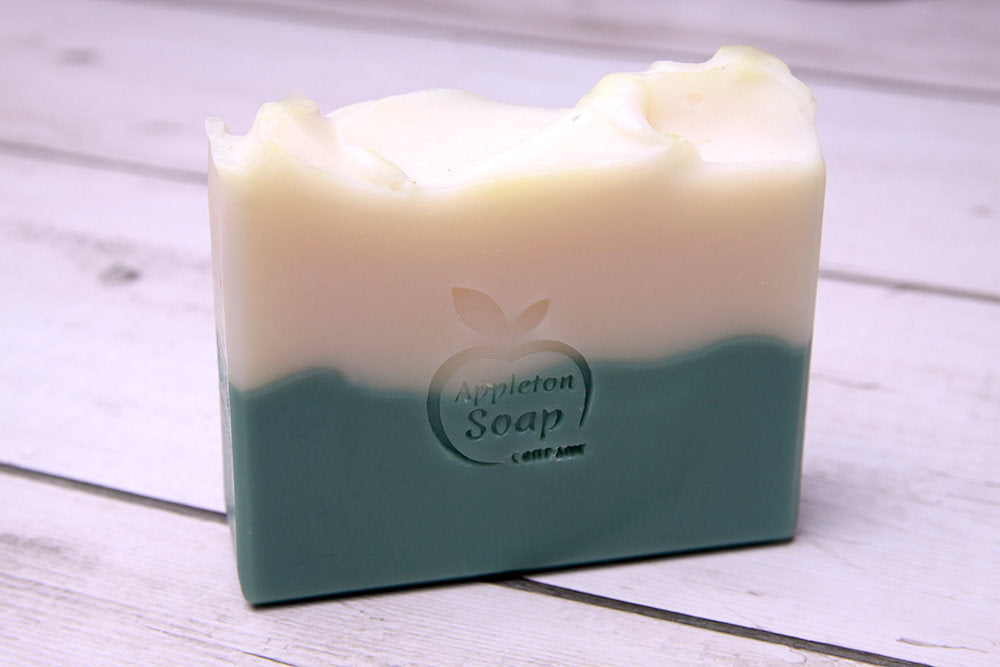Resting on a wide-planked, light-toned wooden surface with visible wood grains, there's a two-toned, rectangular bar of soap. The top half of the soap is a creamy off-white color with brown undertones, while the bottom half is a greyish, teal green. The soap's edges appear chunky and uneven, giving it a rugged, handmade aesthetic. At the center of the bar, there's an engraved logo of an apple with its stem and two leaves, encircling the text "Appleton Soap." Though part of the text is unreadable, the specific and intricate design elements suggest a professional and intentional craftsmanship.